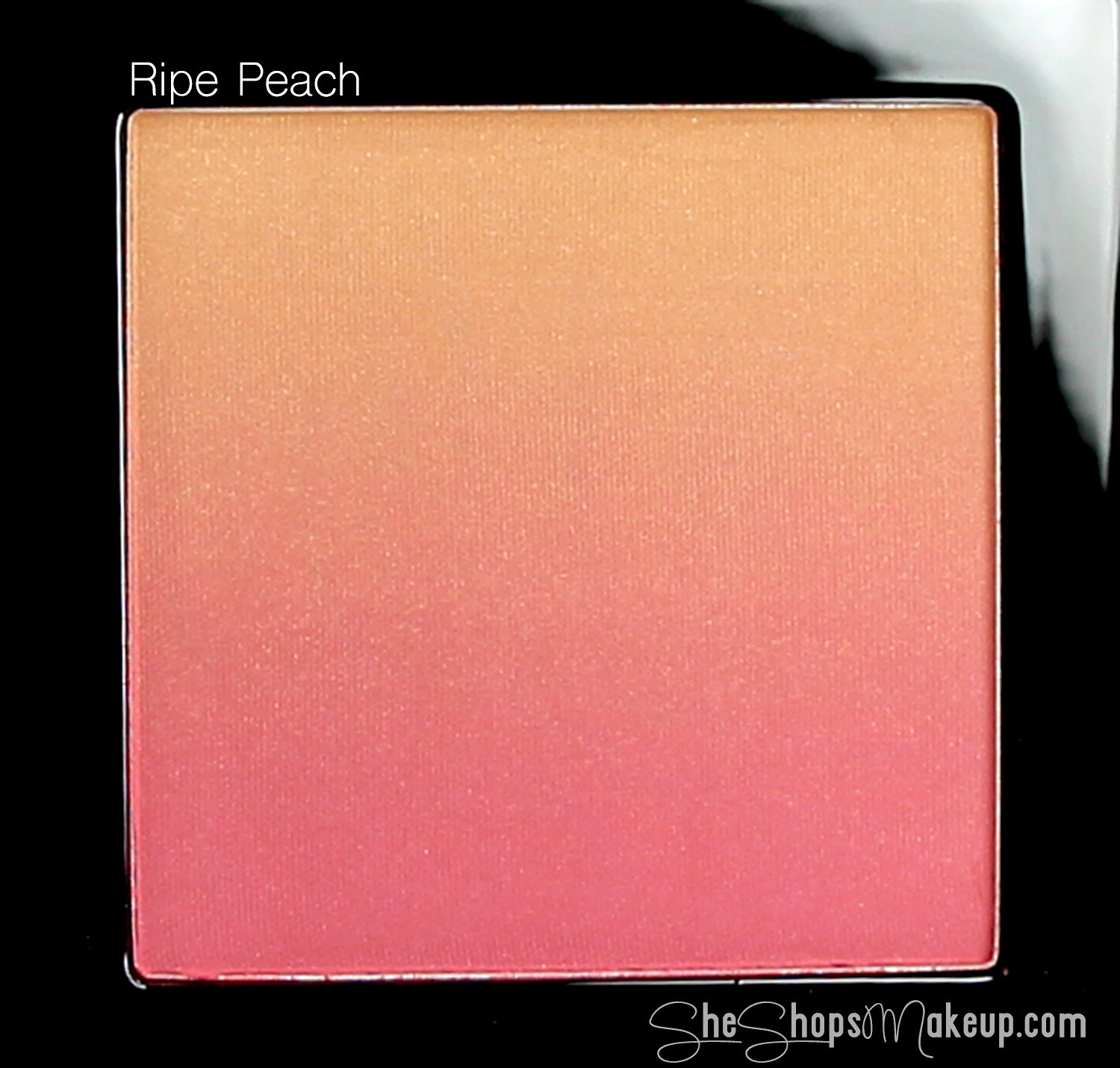This close-up image displays a square container of a versatile makeup product, potentially used as blush, bronzer, or eyeshadow. Set against a predominantly black background, the gradient-toned makeup transitions from a light, gold-ish orange at the top to a soft pink at the bottom. The upper left corner of the image features the product name, "Ripe Peach," in white letters. The lower right-hand corner, also in white, displays the website "SheShopsMakeup.com" with stylized, handwritten-like script for the letters. This image appears to be a professional product display, emphasizing the makeup’s appealing color gradient and sleek packaging.